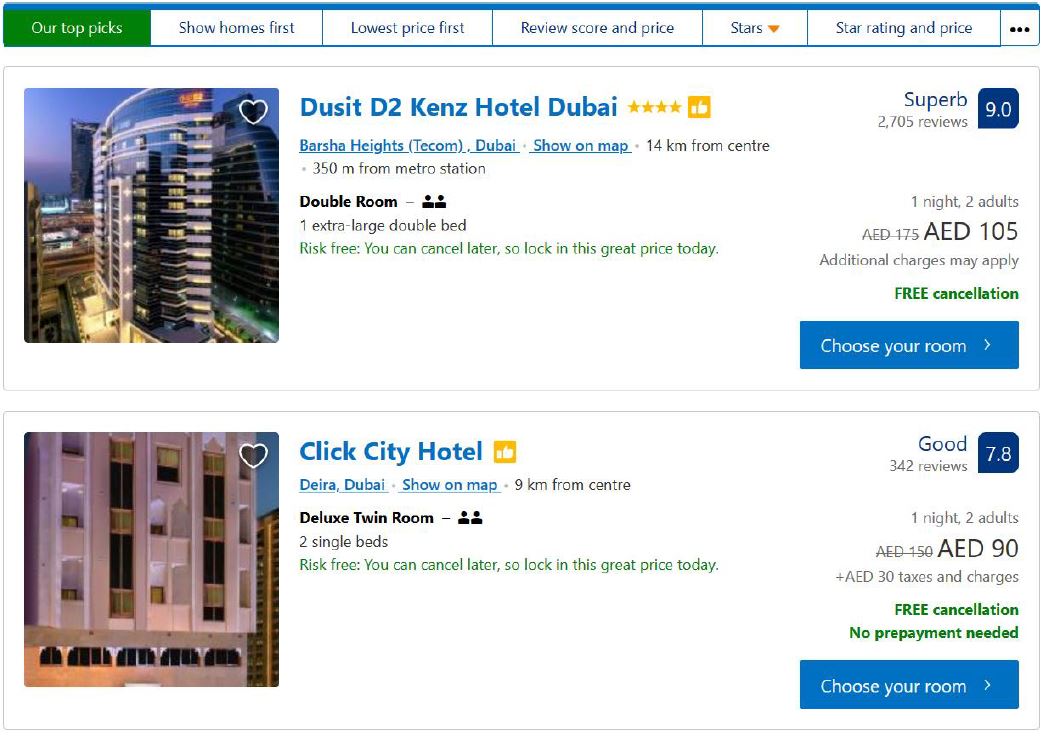**Detailed Caption:**

The image is a screenshot from a travel hotel booking website, displayed in a horizontal orientation. At the top of the screenshot, there is a navigation bar containing six tabs arranged from left to right. The highlighted tab, indicated by a green color, is labeled "Our Top Picks." The subsequent tabs read: "Show Homes First," "Lowest Price First," "Review Score and Price," "Stars," and "Star Rating and Price."

Below the navigation bar are two horizontal content boxes, each bordered by a thin gray line and detailing individual hotel options. The first listing features the "Ducat D2 Kenz Hotel Dubai," with a color photograph of the hotel displayed in a square on the left side. The room rate for this hotel is AED 105, and it boasts a high rating of "Superb 9.0." A blue button labeled "Choose Your Room" is situated below the hotel rating, indicating that this is a risk-free double room option.

The second listing showcases the "Click City Hotel in Deira, Dubai." Similarly, a color photograph of the hotel is shown in a square to the left. The room rate for this hotel is AED 90, with a rating of "Good 7.8." This listing also offers a risk-free room and includes a blue "Choose Your Room" button beneath the rating.